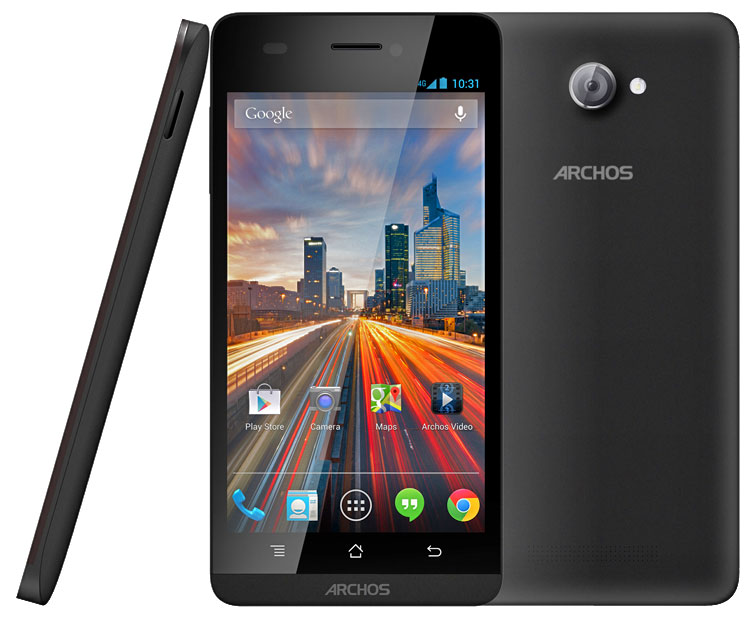This image, likely from an advertisement, features a black Archos cell phone displayed against a stark white background. The photo combines three perspectives of the phone, offering a detailed view from the front, side, and back. On the left, the phone is presented in a thin, sleek side profile, leaning against the frontal view. The front view of the phone prominently displays the Archos branding at the bottom of the screen. The screen itself shows a vivid city skyline with bustling streets, serving as the wallpaper. The top of the screen indicates "Google," the time as 10:31, and a full battery icon. Various app icons, including the Play Store, camera, maps, and Archos video, are visible, along with buttons for phone, chat, news, and a Google browser at the bottom. To the right, the back view of the phone showcases the word "Archos" etched into the surface, accompanied by the camera lens and flash located above the branding. This multifaceted visual effectively highlights the design and features of the Archos cell phone.